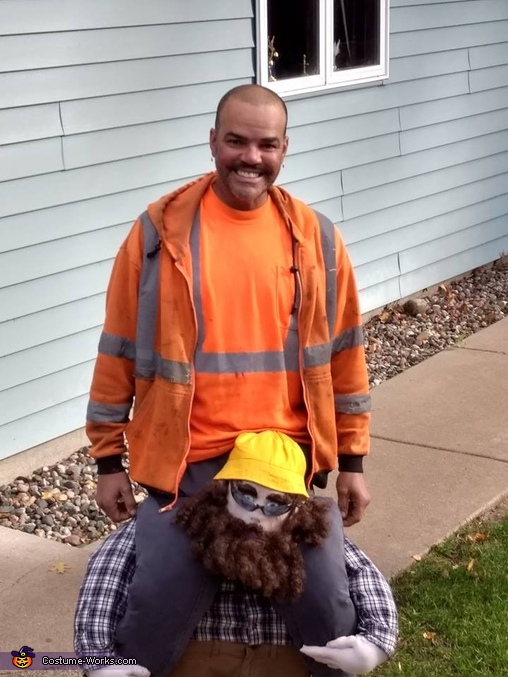The image depicts a joyful man posing in a creative costume, designed to give the illusion that he is being carried on the shoulders of a larger figure. He is facing the camera with a broad smile, donning an orange shirt and an orange construction jacket with reflective stripes. His costume includes dark pants and appears somewhat cumbersome. Below him is a mannequin styled as a bigger, rotund man with a thick curlicue brown beard, wearing a bright yellow hat and sunglasses perched on the bridge of his nose. The dummy, fashioned to look like it's holding the man on its shoulders, has lifelike hands visible with thumb and fingers. The scene is set in front of a neatly maintained, light blue house with white windows, and a well-kept concrete walkway. Adding to the festive atmosphere, there is a small carved pumpkin with a witch hat and a "CostumeWorks.com" label in the lower left corner, suggesting the photo was likely taken for Halloween.